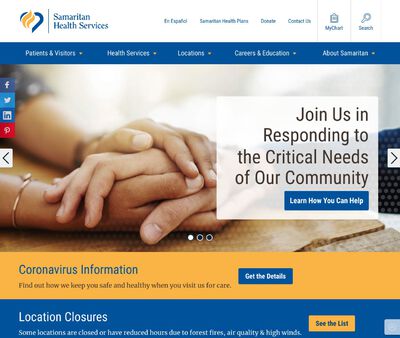The image is a screenshot of the homepage of Samaritan Health Services' website. Predominantly, it features navigation links including "Patients and Visitors," "Health Services," "Locations," "Careers," "Education," and "About Samaritan" situated toward the top of the page. In the top-right corner, there's a login button and a search bar. Central to the homepage is a poignant image of someone holding another person's hand with both hands, accompanied by text urging the community to "join us in responding to the critical needs of our community." Beneath this, a prominently displayed yellow and blue bar provides information on coronavirus, with the yellow section labeled "coronavirus information" in blue text and a "get the details" button in blue. Additionally, there's a segment on "location closures," which includes a brief description and a yellow button. The top-left corner of the page contains quick links to social media platforms like Facebook, Twitter, LinkedIn, and Pinterest. The overall layout appears organized, focusing on essential services and urgent community messages.